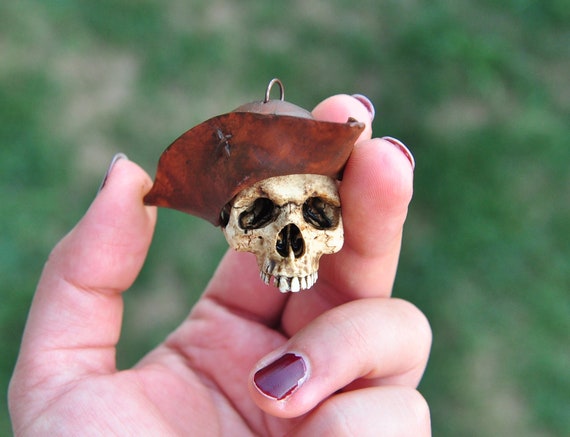In the photograph, a female hand, characterized by its fair complexion and maroon-painted nails, is prominently displayed. The hand is shown palm-up, with the fingers gently cradling a small, aged figurine. The figurine is a weathered skull wearing a brown pirate hat, which is attached to a rusty metal ring, suggesting it is part of a keychain. Detailed textures of cracks and dirt adorn the skull, giving it an antiquated appearance. Notably, the skull lacks its lower jaw, showcasing only the upper teeth, as well as its hollow eye sockets and nasal cavity. The background features a heavily blurred view of a grassy terrain, emphasizing the hand and its intriguing object by creating a stark contrast with the out-of-focus greenery.